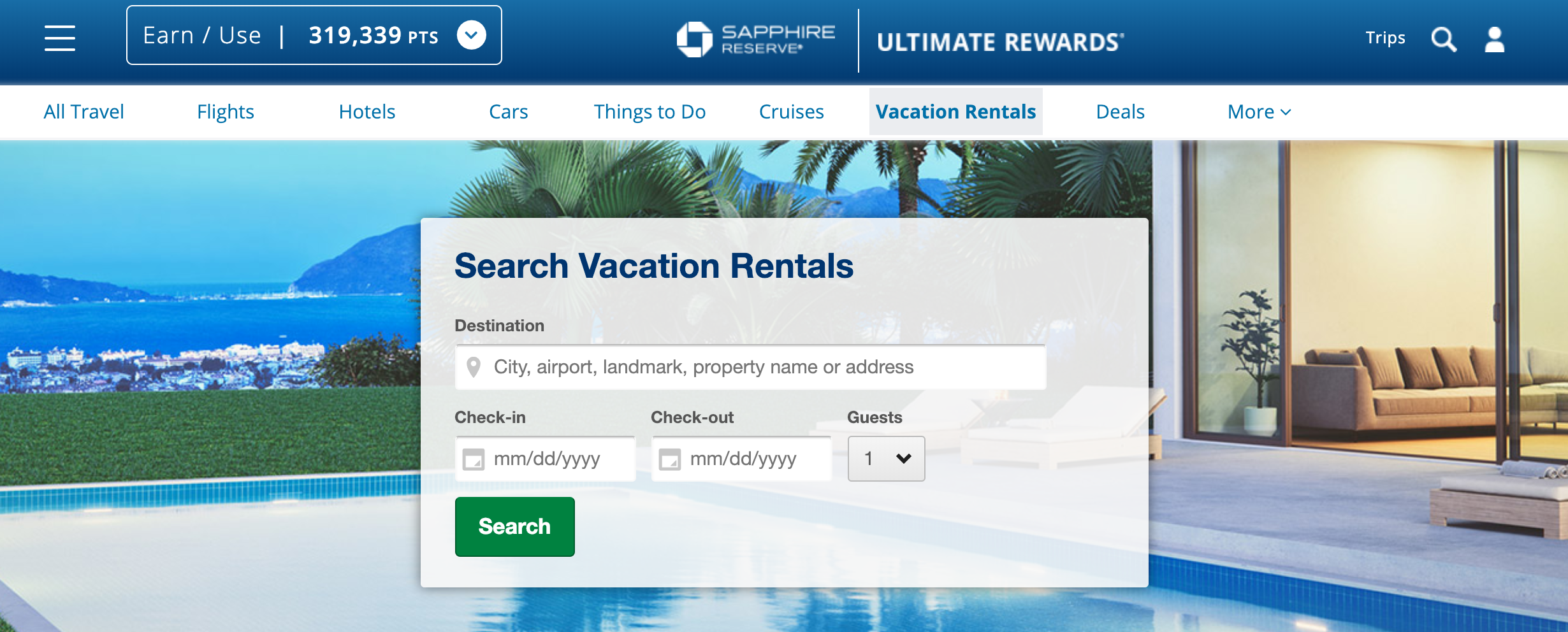A screenshot of a travel website features a blue header bar at the top, containing a hamburger menu on the left and text displaying "earned," "used," and a total of 319,339,000 points. Accompanying these are the "Sapphire Reserve" label and a white logo to the left, with "Ultimate Rewards" positioned to the right of it. At the far right of the top bar are the options "Trips," a white magnifying glass icon, and a person icon, also in white.

Beneath the header, a white navigation bar presents various categories: All Travel, Flights, Hotels, Cars, Things To Do, Cruise, Vacation Rentals, Deals, and a "More" dropdown button. The "Vacation Rentals" category is selected. Below this navigation bar, an inviting image catches the eye, displaying a luxurious swimming pool, a sliding glass window, and a sleek, modern couch inside the adjoining room. In the background, palm trees, serene water, and majestic mountains create a stunning view.

Centrally overlaying this image is a gray search box labeled "Search Vacation Rentals," which includes fields for entering the destination, check-in and check-out dates, and a dropdown menu for the number of guests. At the bottom left corner of this search box, a green "Search" button is prominently displayed.